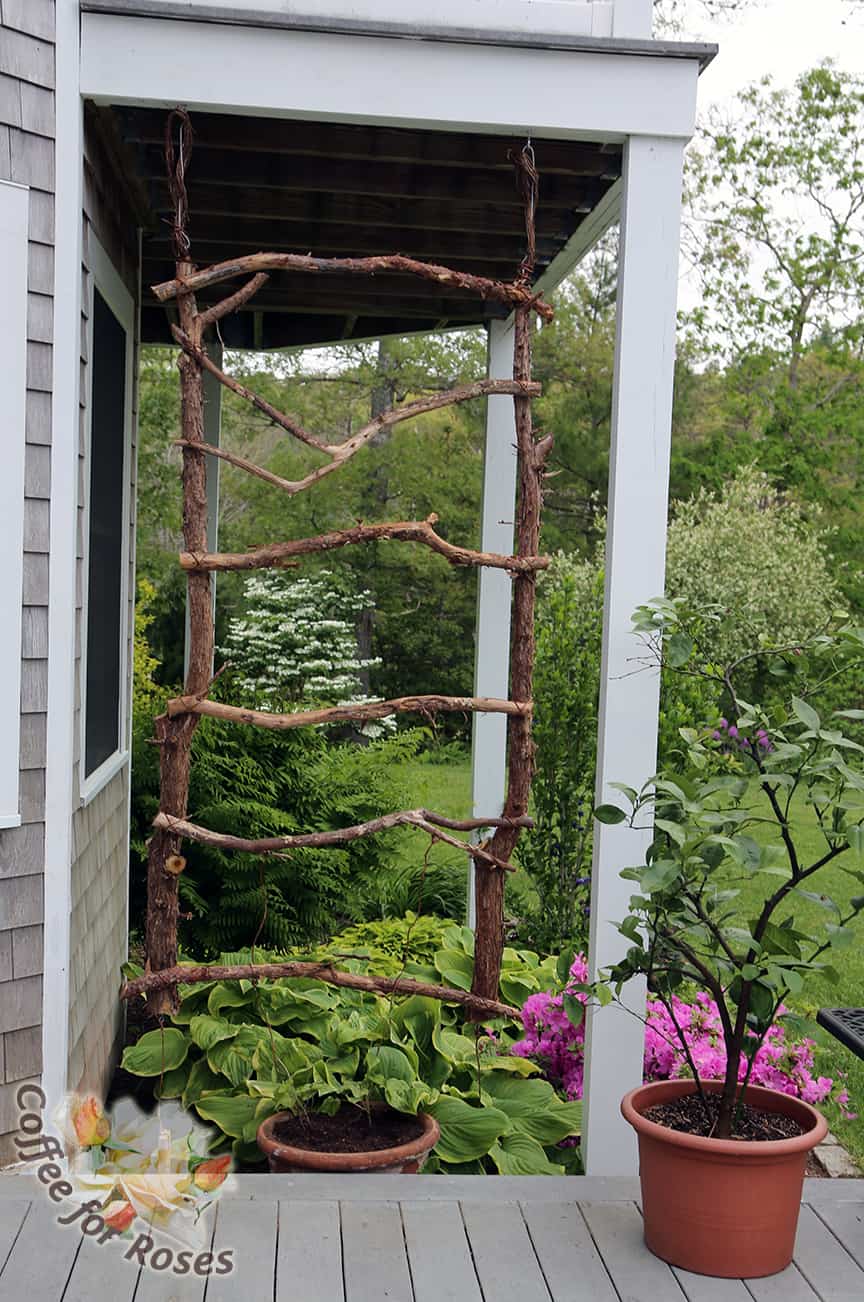In this vertical portrait image, we see the front of a house with grayish tan, shingle siding. Central to the scene is a porch garden with an intriguing natural branch trellis that extends approximately 10 feet high, crafted from tree limbs and sticks. To the left side of the house, under the balcony, are white pillars supporting the structure, adding a classic touch. Below the trellis, there are multiple flower pots; the one on the bottom right contains brown soil with emerging green leaves. Surrounding the porch, a variety of lush green trees and shrubs are present, along with some bushes adorned with pink flowers, possibly rhododendrons. The yard is framed by these plants, creating a vibrant natural setting. In the bottom left corner of the image, a watermark reads "Coffee for Roses," possibly indicating the photographer or a related project. Above, the sky is a muted white, highlighting the greenery of the trees.